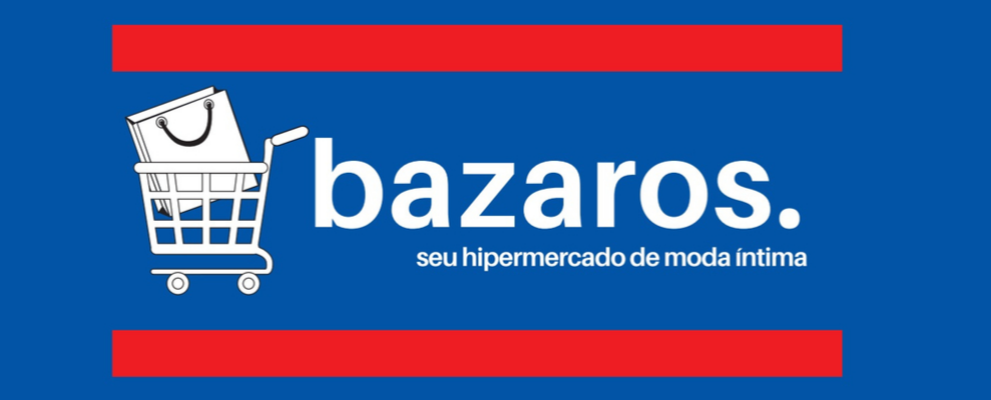The image features a detailed advertisement with a distinct blue background, horizontally framed by two identical red bars at the top and bottom. Prominently, a shopping cart in white is positioned on the left side, within which sits a shopping bag, also in white with a black handle. This handle creates an impression almost like a smiling face. To the right of the cart, in white text, is the word "Bazaros" followed by a period, seemingly the store's name. Below this, it reads "Su Hypermercado De Moda Intima" in Spanish. The sign carries an aura of a hypermarket or an online shopping advertisement, possibly targeting a Spanish-speaking audience.